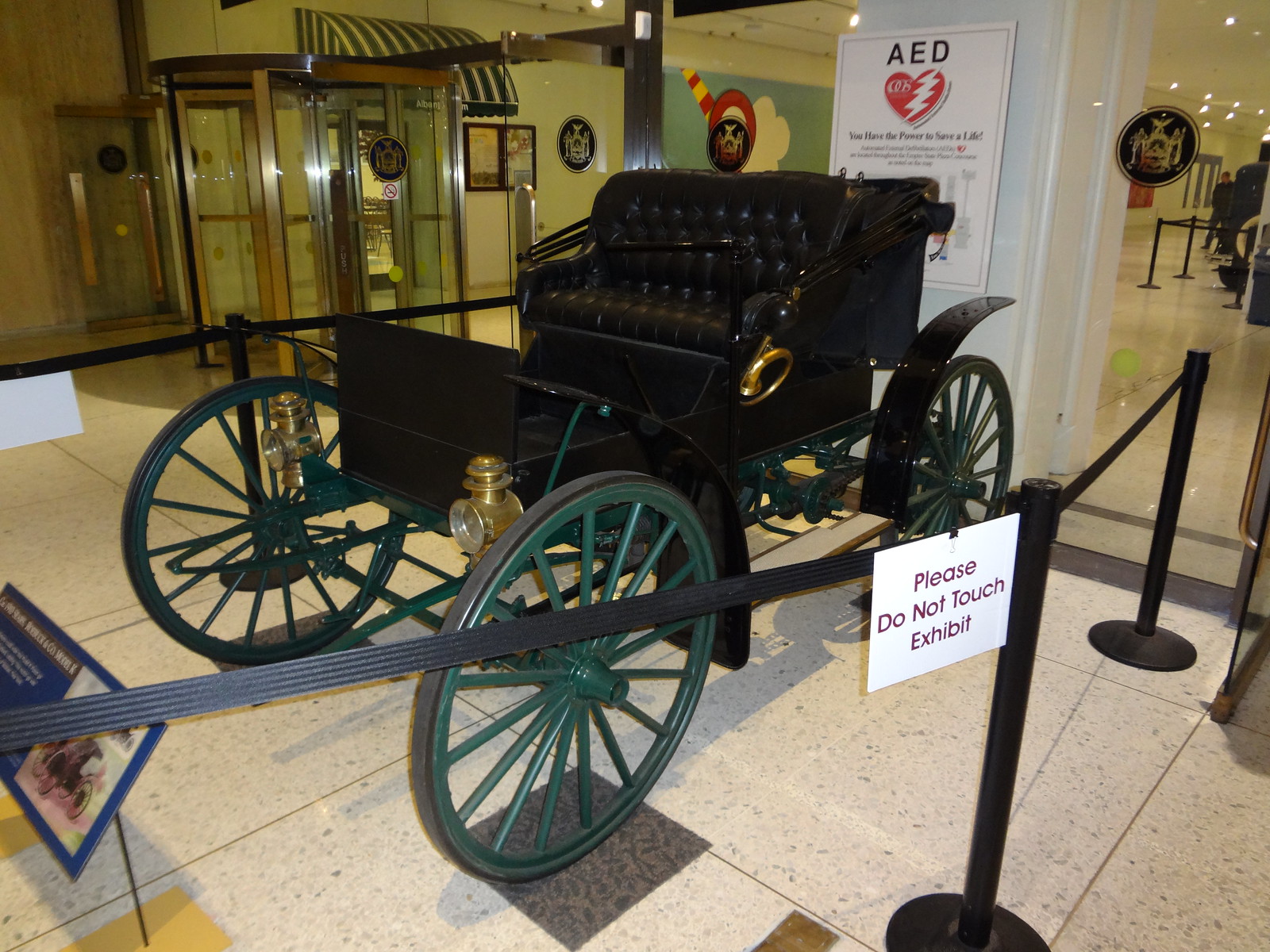This image captures a detailed, historical exhibit of an old-time open-top carriage prominently displayed in a museum-like setting. The carriage features a black front and black leather seats, designed for two people. It is equipped with green spoked wheels, resembling traditional wagon wheels, which are about two feet in diameter. The four wheels have black fenders, and two lanterns are mounted above the front wheels. The vehicle appears to have a convertible roof, hinting at its antique design meant to be horse-drawn.

The exhibit is carefully roped off with four posts connected by a black belt, marked with a sign that reads "Please do not touch the exhibit." In front of the carriage, there is a blue stand containing image and text details about the carriage, though they are too far away to be legible. Behind this stand, a white column bears an AED sign, featuring a red heart with a white lightning bolt and accompanying text too small to read.

The background reveals a glass wall through which people can be seen queuing, possibly at a pay station. Farther back, about 20 or 30 feet, one can see the museum entrance with a white glass door. The walls surrounding the door are light green, adorned with circular seals and designs, contributing to the historical ambiance. To the right, a blue wall displays a cloud and a figure within a red circle, adding further context to the museum's thematic elements.